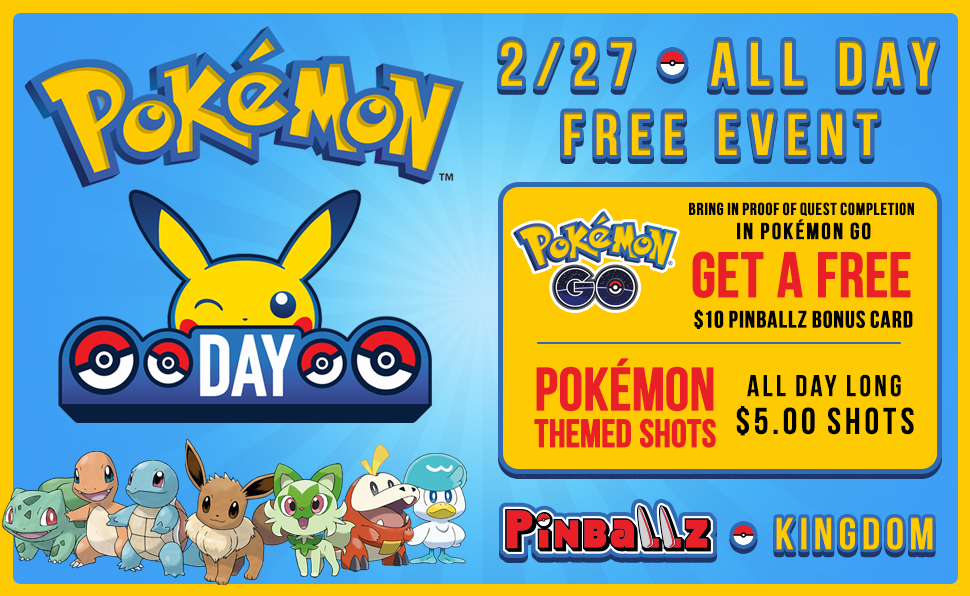Here's a revised and detailed caption for the image:

---

This image is an advertisement for "Pokemon Day," presenting as a vibrant rectangular poster. The poster is bordered in bright yellow, with a light blue background that creates a playful and inviting ambiance. On the left side, the iconic "Pokemon" text is prominently displayed in its characteristic yellow and blue font. Directly below, a small blue banner reads "Day," flanked by two Pokeballs on either side and featuring a winking Pikachu peeking over the edge, adding an element of charm and nostalgia.

Below the banner, a delightful assembly of Pokemon characters is depicted, including some familiar faces such as Bulbasaur, Charmander, Squirtle, and Eevee. Additionally, there are three other Pokemon on the right side whose identities are not specified.

On the right side of the poster, important event details are provided at the top. The text announces "2.27 All Day Free Event," indicating the date and free entry. The advertisement specifies a special promotion for Pokemon Go players: "Bring in proof of quest completion in Pokemon Go, get a free $10 Pinballs Bonus Card." This suggests integration with the popular mobile game to enhance attendee engagement.

Moreover, highlighting the event's fun and festive atmosphere, it mentions "Pokemon-themed shots all day long" available for $5 each. The event is associated with "Pinballs Kingdom," as indicated by the red text and accompanying Pokeball symbol at the bottom of the poster.

Overall, the poster promotes a lively Pokemon-themed day, likely hosted at a bar or entertainment venue, featuring drink specials, game-related promotions, and an exciting community gathering for fans of all ages.

---

This caption provides a comprehensive and vivid description of the event and the poster's layout.